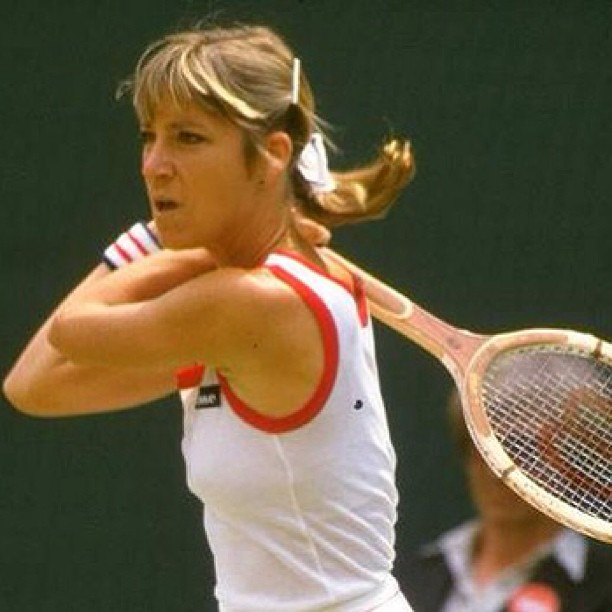The image captures a professional female tennis player in mid-action, possibly during a professional match rather than a practice session. She is depicted from the waist up, poised in an action stance, seemingly in the aftermath of a powerful serve. Her intense expression and open mouth suggest the concentration and effort put into her play. She holds a wooden racket behind her back with both hands. The player sports a white tennis outfit, consisting of a white shirt with red accents around the neck and arms, paired with a white skirt. 

Her blonde hair is pulled back into a ponytail, secured with barrettes and a white bow, blowing slightly in the wind. An armband with red, white, and blue stripes adorns her right wrist. The background features a blurred woman, probably a line judge, dressed in a dark blazer and white button-down shirt, indicating the professional setting of the match. The colors in the photograph include various shades of tan, peach, brown, black, white, red, and navy blue, and the setting appears to be an old stadium with green surroundings.